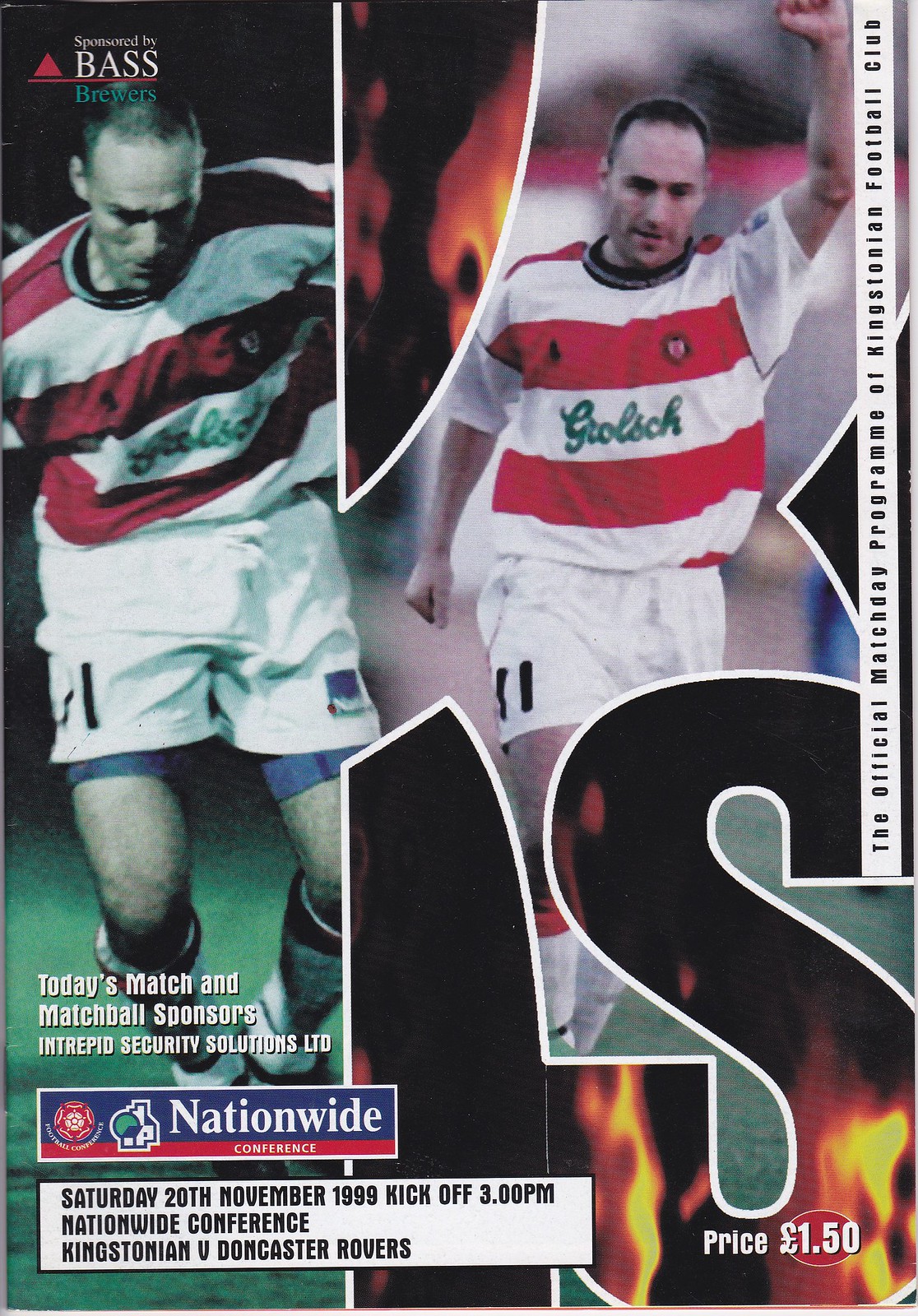This detailed cover description captures the sports theme and key elements consistently mentioned by all three sources.

"The cover of the official match day program of the Kingstonian Football Club is prominently marked by a large white outline of a red 'K' with a small 'S' at the bottom right of the 'K'. The cover features two male soccer players dressed in red and white striped jerseys and white shorts, one with his hand raised and the other looking down. The program is sponsored by Bass Brewers and has a vertical white bar on the right side with black vertical text reading 'The Official Match Day Program of Kingstonian Football Club.' Additionally, it indicates 'Growlish' on the jersey and highlights Intrepid Security Solutions Limited as the match ball sponsor. The program is priced at £1.50 and covers the Nationwide Conference, with details of the match between Kingstonian and Doncaster Rovers on Saturday, 20th of November, 1999, with a kickoff at 3 p.m. A background of flames and black within the 'S' adds to the dynamic design."